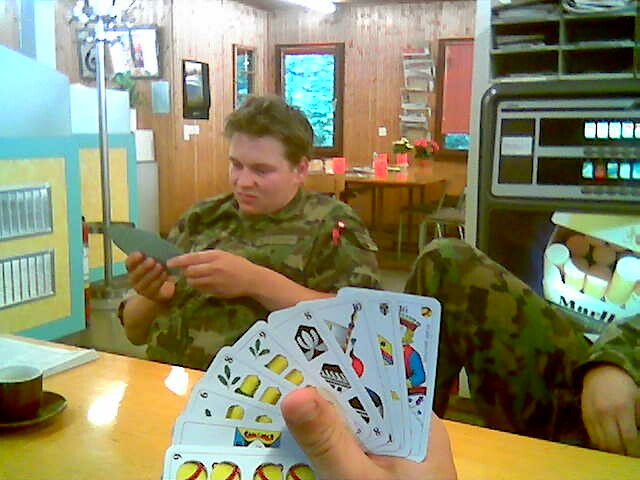The image depicts a scene involving at least two, possibly three, individuals donned in army fatigues with rolled-up sleeves, engaged in a game of cards. The cards are distinctive with a design that includes depictions of lemons, candles, or possibly a king, and exhibit vibrant colors – white background with yellow, red, and blue details. The setting includes a simple brown laminate table occupied by a brown coffee cup on a saucer, a sheet of paper in front of one individual, and a cigarette machine just beyond another man with a knee up. This cigarette machine features a prominent yellow sign with marble patterns and grayish lines beneath the buttons. In the background, another brown table, gray chairs, and a reddish-brown window frame are visible, along with a two-partition wall colored teal-blue and yellow, adorned with silver vents, creating a vivid and dynamic backdrop.